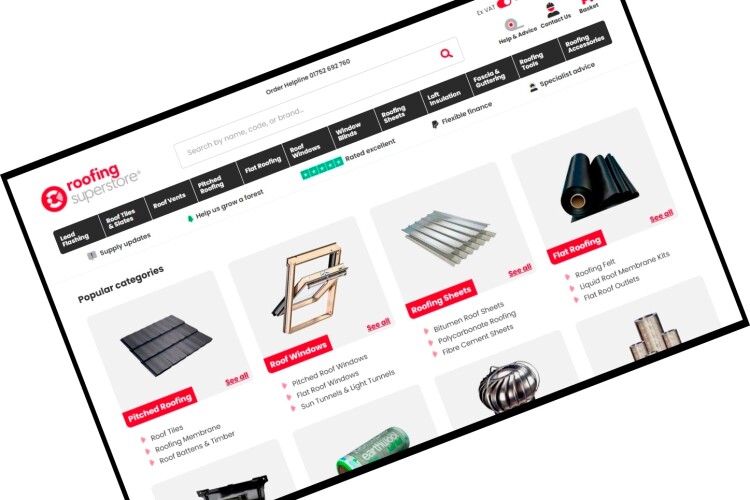The webpage for Roofing Superstore features a prominently displayed header with "Roofing" in red font and "Superstore" in grey. The site's logo is on a red background with white and red accents. A search field invites users to "search by name, code, or brand," complemented by an order helpline with a listed phone number. Key navigation buttons include "Help and Advice," "Contact Us," and "Basket."

The main navigation bar provides tabs for various categories, such as Lead Flashing, Book Tiles and Slates, Roof Ventilation, Pitched Roofing, Flat Roofing, Roof Windows, Window Blinds, Flooring Sheets, Loft Insulation, Roofing Tools, and Roofing Accessories. Below this, users will find a "Supply Update" button and an initiative button labeled "Help Us Grow a Forest," featuring a tree icon.

Customer rating is highlighted with a five-star "Rated Excellent" badge on a green background. Popular categories are visually represented with images: Pitched Roofing shows a grey hue, Roof Windows in a wooden finish, Roof Sheets in silver, and Flat Roofing in black. The overall design uses a white background with black text and intermittent red icons for accents.